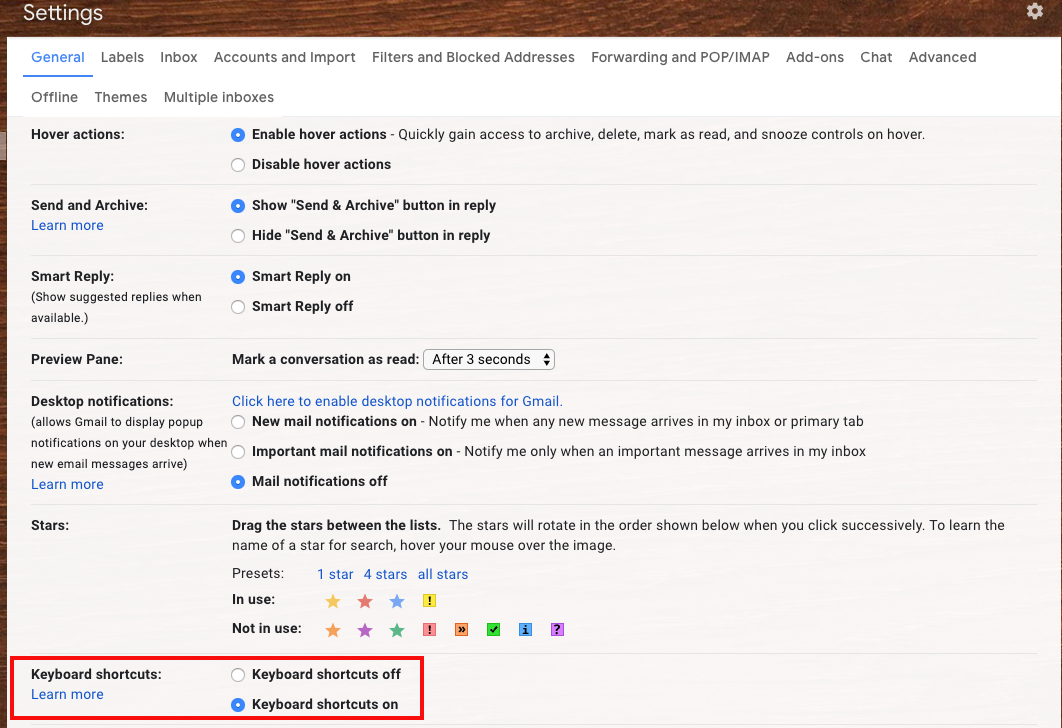The web page features a "Settings" label prominently displayed in the upper left-hand corner, embedded within a dark brown ribbon that spans the top of the screen. This ribbon is designed with a wood grain texture, giving it the appearance of a piece of dark wood. Directly beneath this ribbon, on a clean white background and running horizontally from left to right, are various tabs labeled "General," "Labels," "Inbox," "Accounts and Import," "Filters and Blocked Addresses," "Forwarding and POP/IMAP," "Add-ons," "Chat," and "Advanced." Below this row, additional tabs labeled "Offline," "Themes," and "Multiple Inboxes" are displayed.

The "General" tab is highlighted in bright blue with an underline, indicating it is currently selected. The majority of the page below this section features a light blue background, populated with a vertical list of categories written in black text. These categories include "Hover Actions," "Send and Archive," "Smart Reply," "Preview Pane," "Desktop Notifications," and the final category, "Stars." To the right of each category in this list, various configuration options are available for the user to adjust settings accordingly.